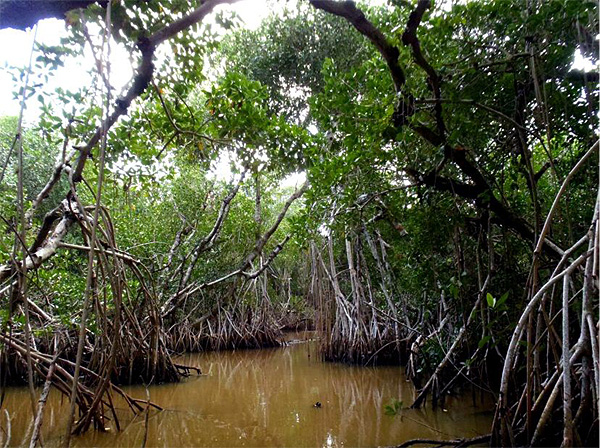This photograph captures a reflective scene reminiscent of a Louisiana bayou. The foreground features a swampy, muddy waterway that winds through the center and extends into the distance, bordered by weathered and dried clusters of branches and sticks emerging from the water. The water itself is a murky light brown, accentuated by streaks of white reflections from the overhanging tree branches. On either side of the waterway, dense brush and green trees frame the scene, their foliage transitioning from green at the top to brown at the base. Notably, on the left, a prominent white branch juts into the water, with smaller, thinner branches hanging down. The right side is populated mostly by these smaller branches. Above the swamp, white clouds fill the sky, with a patch of blue visible in the upper left corner. Reeds rise vertically from the water along the narrow path, contributing to the dense and intricate natural tapestry. The overall scene exudes a sense of stillness and quietude, permeated by the rich textures of natural growth and decay.